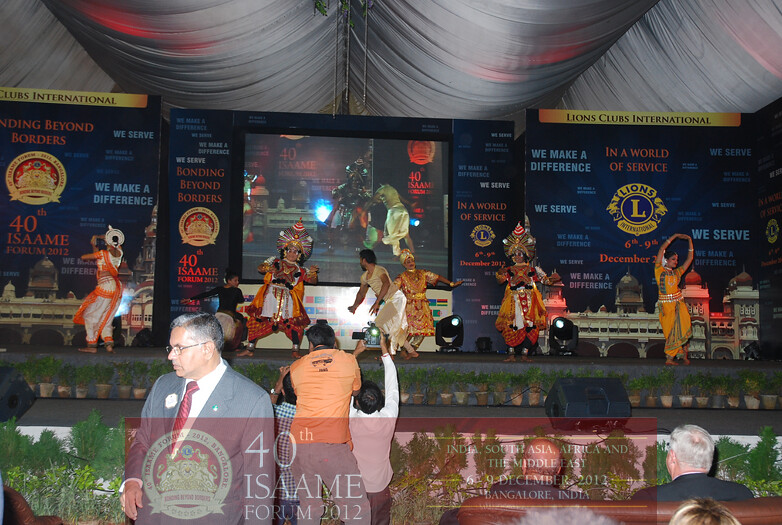The image captures a vibrant cultural performance at the 40th ISMI Forum, held in December 2012 in Bangalore, India. A diverse group of 5 to 7 dancers is on stage, adorned in elaborate traditional attire that features rich hues of yellow, orange, red, and black. Both men and women showcase their heritage through intricate costumes, with men wearing ornate gold headdresses and women in elegant yellow dresses. The stage is surrounded by small potted plants in red clay pots, adding a natural touch to the setting.

Behind the dancers, a large digital screen broadcasts the performance to the audience, ensuring visibility for all attendees. Additional signage includes banners with phrases like "Lions Club International," "We Make a Difference," and "We Serve," highlighting the event's affiliation and mission. The audience is visibly engaged, with some members enthusiastically clapping and others capturing the moment with cameras. The ceiling above is composed of large gray horizontal cylinders, contributing to the overall structural ambiance of the event.